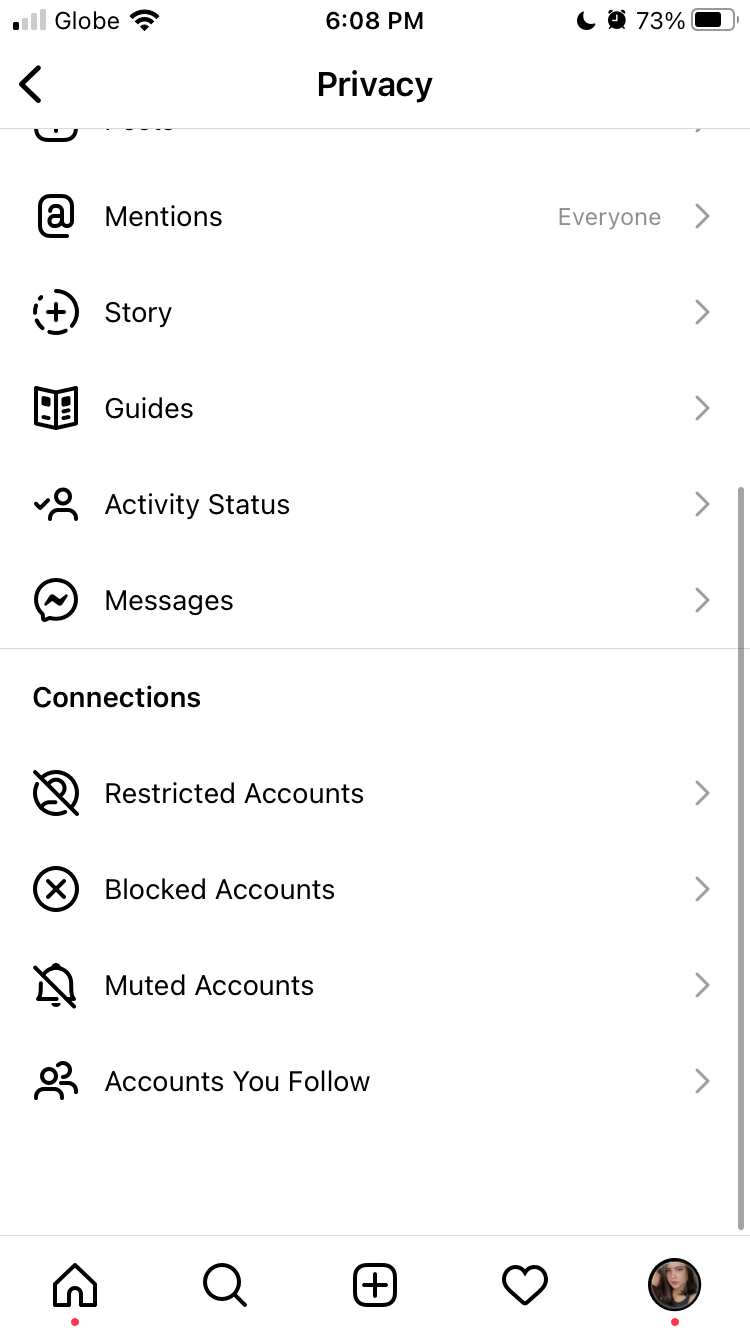The screenshot from a smartphone or tablet displays various features and settings. On the top left corner, it shows a weak signal strength indicated by 1 bar out of 4, followed by the carrier name "GLOBE" with a capital "G." Next to it, a fully connected Wi-Fi signal icon is shown. 

Centrally positioned is the time "6:08 PM," adjacent to which are a crescent moon icon, signaling Do Not Disturb mode, a black clock icon, and a battery symbol with a charge level of 73%.

Further down, a black arrow pointing left signifies a back button. In the middle of the screen, "PRIVACY" is labeled in large, capitalized text on an off-gray, almost light gray, background. Below this, partially visible at the bottom, is a square with a cursive "A" labeled "MENTIONS" on it.

On the right side, the word "EVERYONE" appears in gray text accompanied by a gray arrow. Multiple sections follow, each with descriptive icons. A dotted circle with a plus sign labeled "STORY" is present, which starts to fill up. Nearby, there's an icon resembling a newspaper for "GUIDES." Below that, a circle with the silhouette of a person and an overturned half-circle with a checkmark labeled "ACTIVITY STATUS" appears, with the checkmark on the left.

Additionally, a circle with a squiggly line labeled "MESSAGES" suggests Facebook Messenger functions. Underneath this is a bold subheading "CONNECTIONS," with several account management options presented below. These include:

- A circle with a silhouette of a person and a line through it, labeled "RESTRICTED ACCOUNTS."
- A circle with an X, labeled "BLOCKED ACCOUNTS."
- A bell icon with a line through it, labeled "MUTED ACCOUNTS."
- Two overlapping silhouettes of people labeled "ACCOUNTS YOU FOLLOW."

This detailed view provides a comprehensive understanding of the various settings and notifications available on the device.